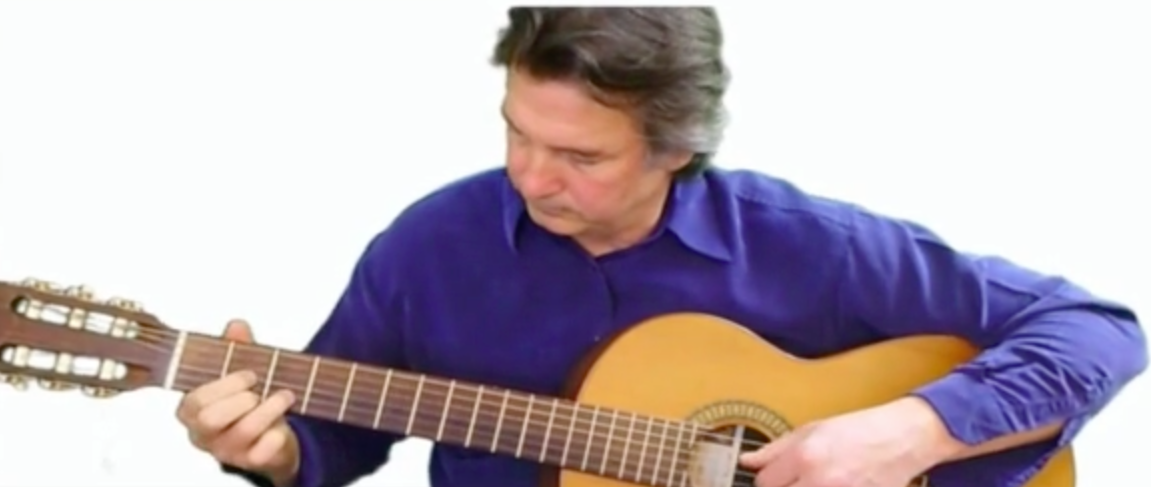In this somewhat blurry image, a middle-aged man with salt and pepper, medium-length hair that grows over his ears, is captured playing an acoustic guitar. He is clean-shaven and dressed in a purplish-blue collared button-down dress shirt, with its sleeves unbuttoned and loose at the wrists. The man is seated against a plain white background, looking down at the neck of his light brown acoustic guitar, which features a darker brown neck and silver-colored strings. His right hand is near the neck of the guitar, with fingers positioned on the strings, while his left hand is placed near the base, strumming. Though the photo appears grainy, it evokes the sense of a candid moment, potentially from a guitar lesson video.